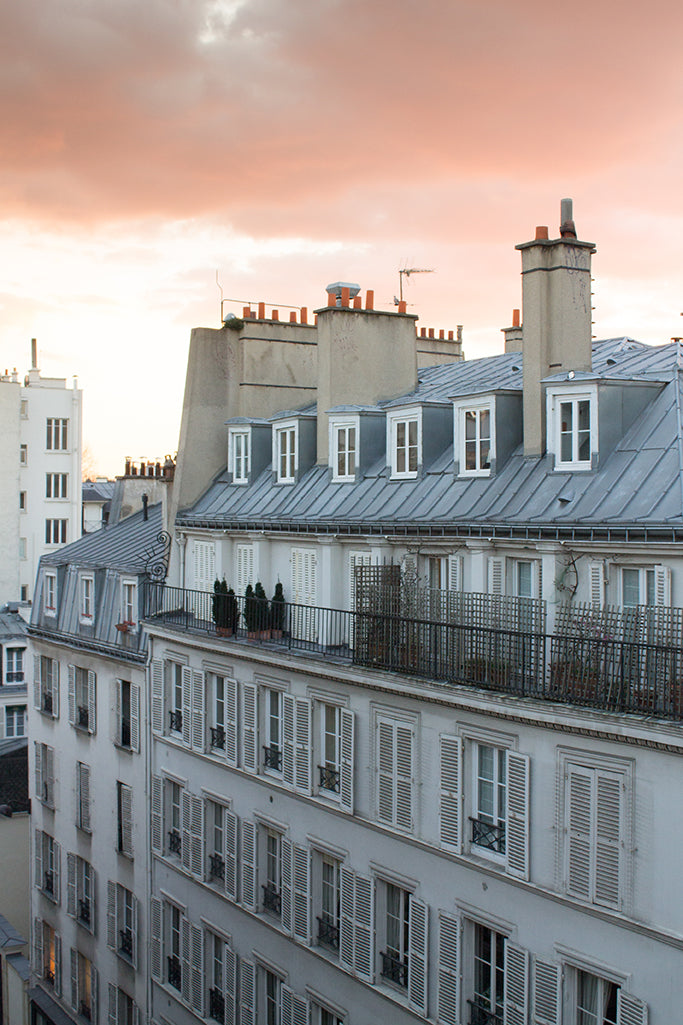The photograph is a portrait layout depicting an outdoor scene dominated by a tall, white multifamily building, possibly a hotel, with numerous windows and shutters—some adorned with gates. The building features a light blue to gray roof contrasting against its primarily white sides. The sky occupies the top third of the image, presenting a cloud-covered, pink-hued atmosphere that suggests early morning or late evening light. The background reveals additional white buildings, adding depth to the urban setting. In the lower left-hand corner, light shines through two windows, indicating activity within the building. The image is clear and bright, thanks to the ample natural light, and contains no text, numbers, or extraneous elements.